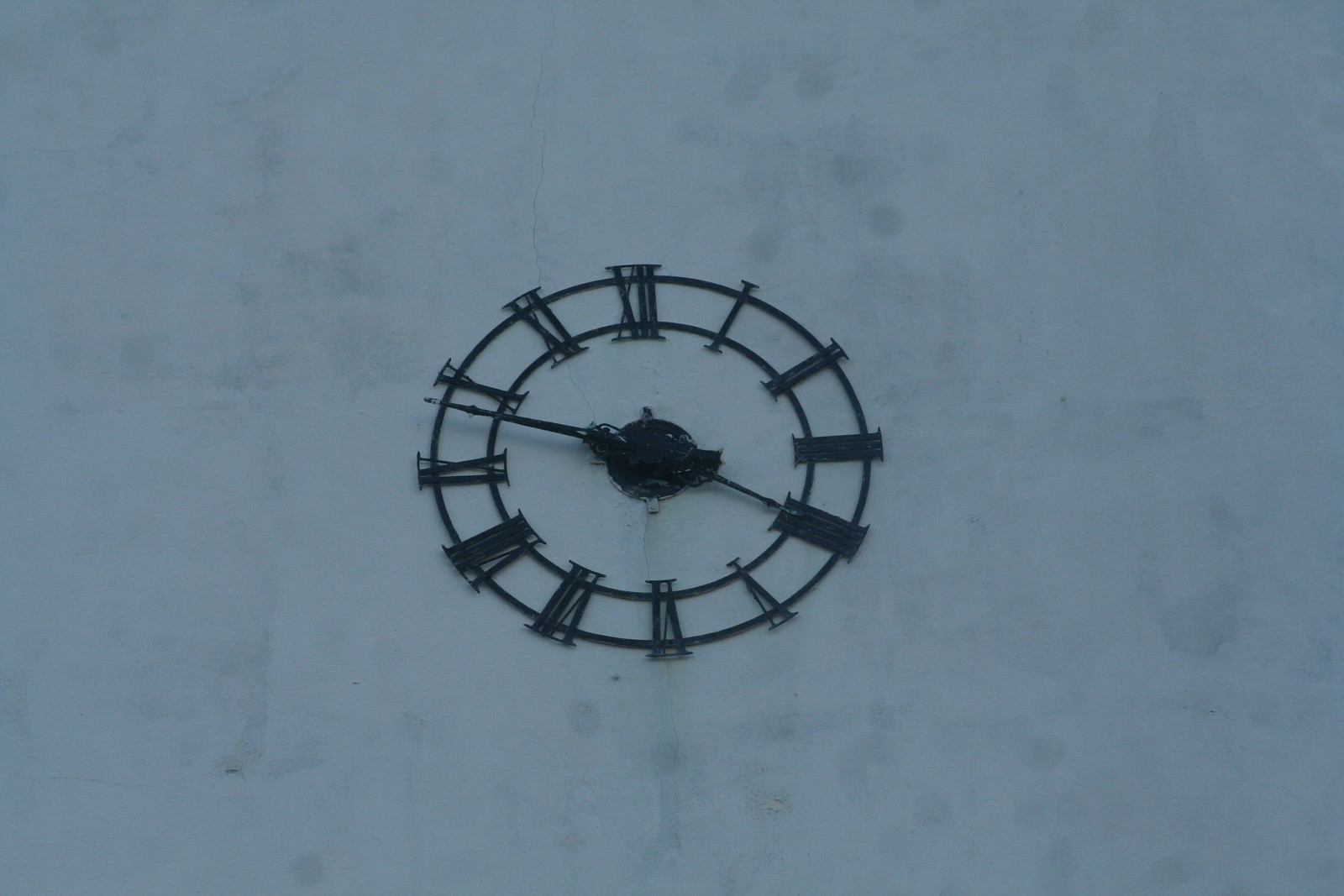The photograph features a rectangular composition with its longer sides at the top and bottom and shorter sides on the left and right. At the center of the image is a clock affixed to a tall, gray concrete wall, which is marked with various dark gray spots, evidencing wear or natural imperfections in the material. The clock itself is designed with two concentric black circles that are connected by Roman numerals to indicate the hours. Starting from the top, the numerals read X-I-I (12 o'clock), followed by I (1 o'clock), I-I (2 o'clock), and I-I-I (3 o'clock). Two black hands extend from a central black circle, the longer one indicating the minutes and the shorter one denoting the hours, reflecting the traditional timekeeping design. The stark contrast between the black elements of the clock and the gray tones of the concrete wall contributes to the industrial and robust aesthetic of the photograph.